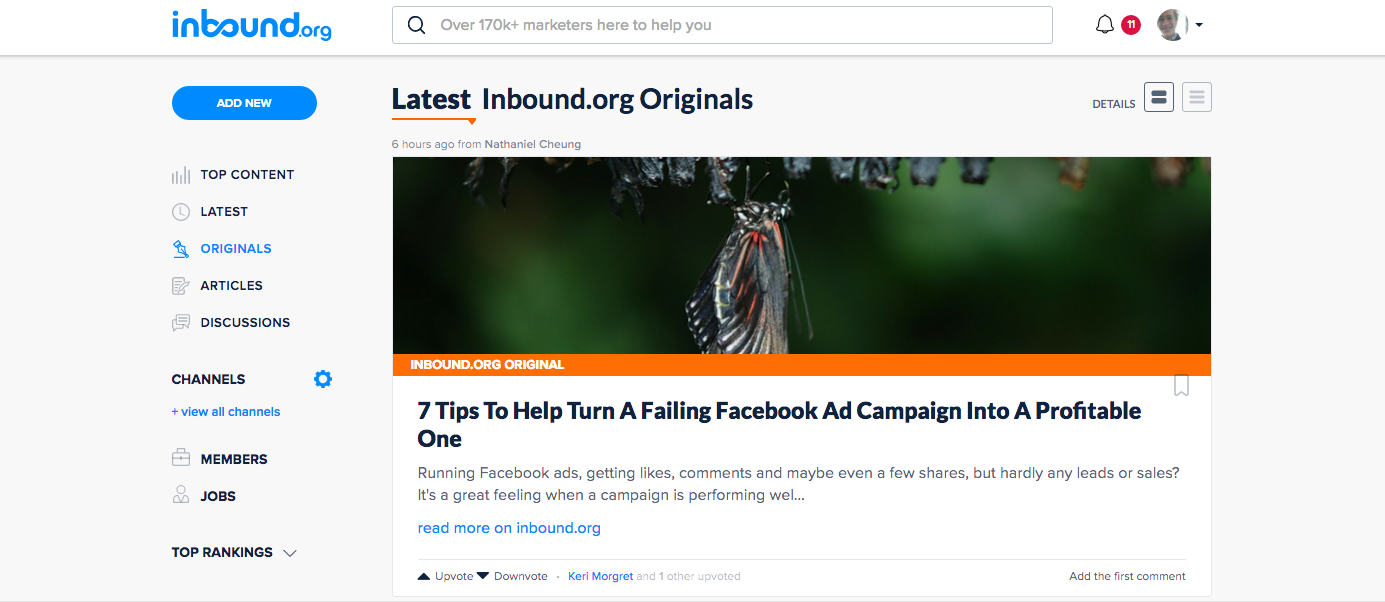Sure, here is a cleaned-up and detailed descriptive caption:

---

The image showcases a webpage from inbound.org. At the top, there is a prominent white bar stretching across the width of the page, creating a clean header section. Below the bar, the page background transitions into a light gray hue. 

Centered within the white bar is the word "Inbound" in a striking blue font. Just beneath, a large search bar is prominently displayed in the top center, accompanied by the text "Over 170,000 marketers here to help you," conveying the community-driven nature of the site. 

On the top-right corner, there is a notification bell icon with a red dot next to it, indicating the presence of unread notifications. Nearby, a profile picture of the user is visible, marking easy access to personal account settings.

To the left of the search bar, there is a blue button labeled "Add New" in white text, inviting users to contribute new content or initiate actions on the site.

Below the header, a horizontal list of tabs is displayed, featuring categories such as Top Content, Latest, Originals, Articles, Discussions, Channels, View All Channels, Members, Jobs, and Top Rankings, facilitating easy navigation through the site's extensive content.

In the main content area, centrally placed, there is a headline reading "Latest inbound.org Originals," catching the user's attention. Beneath this header, a visually appealing image of a butterfly is accompanied by a featured article titled "Seven Tips to Help Turn a Failing Facebook Ad Campaign into a Profitable One." Additional details and information about the article are displayed below this title.

---

This caption provides a comprehensive and visually descriptive narration of the webpage, highlighting its structure, key elements, and functionalities.